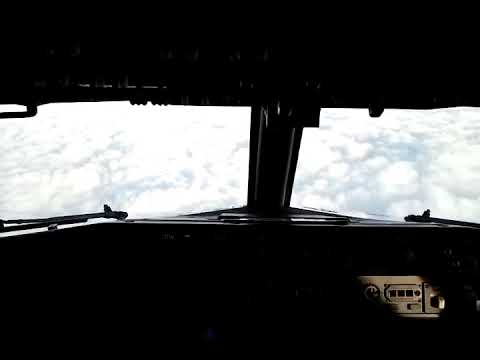The image is a rectangular photograph, approximately four inches wide and three to four inches tall, taken from within an airplane cockpit. The top and bottom thirds of the image are mostly in darkness, framing the view through the cockpit's windows. Between the windows, separated by a vertical black strip, the scene outside reveals a stunning expanse of fluffy white clouds with patches of blue sky, indicating the airplane is flying above the cloud layer. The cockpit itself is very dark, making it difficult to distinguish specific details, except for a faintly visible section of the control panel in the lower right corner. This panel features three small buttons, a knob, and possibly a switch, illuminated by a beam of light coming from the upper left corner. Additionally, windshield wipers and overhead handles, possibly part of the throttle system, can be subtly discerned amidst the shadows.